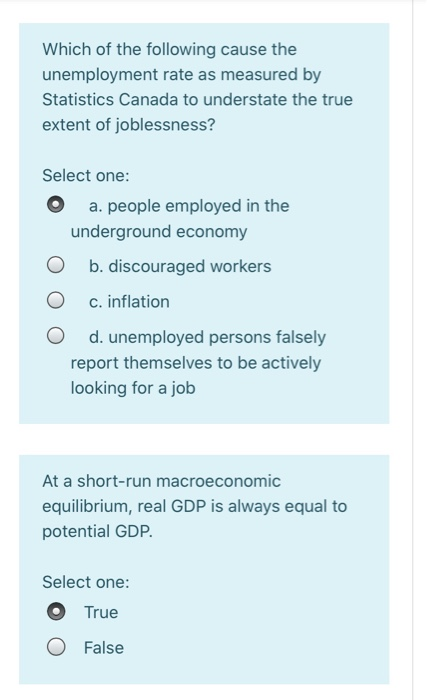This image is a cropped screenshot of an online economic assessment. The screenshot features a small, thin gray bar at the top, which extends over to the right, indicating that part of the right section is also cut out. The screenshot's left, bottom, and additional right sections have been cropped, leaving only a portion of the original image visible. 

Within the image, there are two distinct blue boxes, each with a light blue background. The upper box is notably larger than the lower one. Both boxes contain economic-related questions accompanied by instructions to "select one" response. 

In the top box, four possible answers are listed, with the first option (A) selected. In the smaller, lower box, a true/false question is presented, and "True" has been selected. This composition suggests that the screenshot is from an interactive online platform designed for an economic assessment.